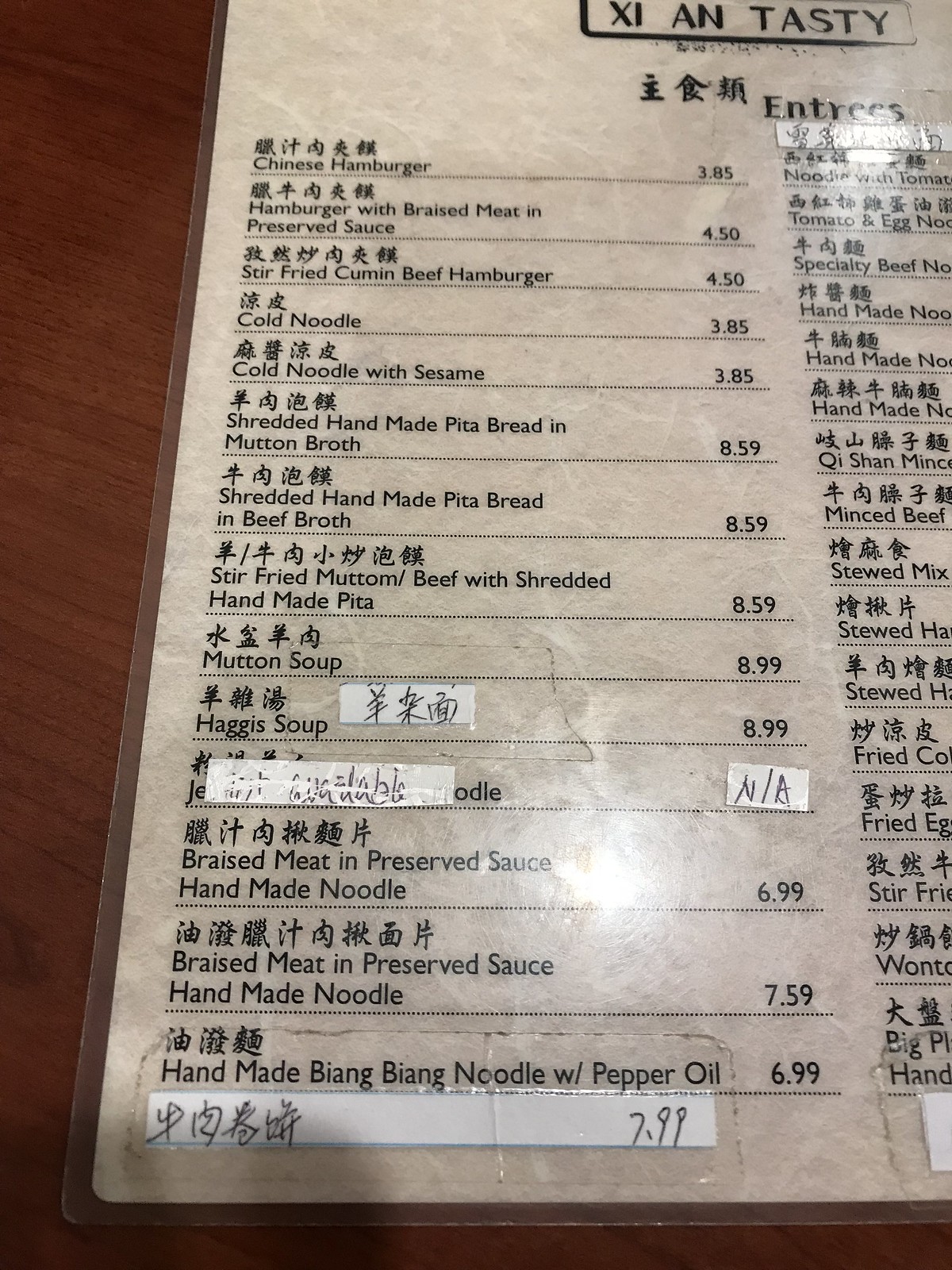The image captures a laminated menu resting on a wooden-grain surface. The menu itself is white with black text and features both a foreign language, presumably an Asian script, and English translations. The text is clearly legible under the bright overhead lighting, which causes reflections on the menu's glossy surface. The content is organized with entrees listed on one side, showcasing their names and descriptions in the foreign language followed by English explanations, along with the corresponding prices in English. Notably, some items on the menu have been modified using white tape – one item has been covered to indicate it's no longer available, while another has a hand-written addition on white tape. The image reveals approximately three-fourths of the menu, with the bottom left corner cut off, revealing that the menu is positioned diagonally to the right. The second column, which likely continues the list of entrees, is partially obscured.